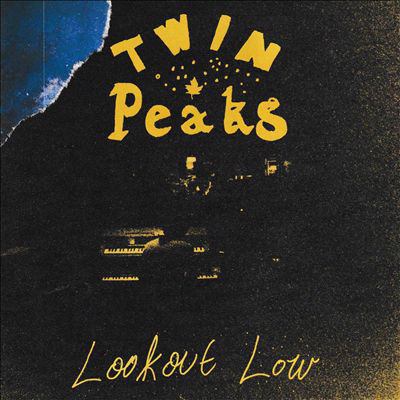The image is a dark, grainy album cover featuring a blurry scene that appears to have been captured on stage. Dominating the image is a man sitting at a piano or organ, positioned near the lower left. The surrounding objects and background are difficult to discern due to the darkness. The text "Twin Peaks" is prominently displayed at the top in yellow with a small yellow maple leaf and dotted embellishments. Positioned at the bottom in cursive, the words "Lookout Low" are also in yellow. The top left corner of the image gives the impression of a torn photograph, revealing a patch of blue sky. The overall aesthetic, marked by its old, faded, and somewhat damaged appearance, hints at it being the front cover of a vintage CD or vinyl record.